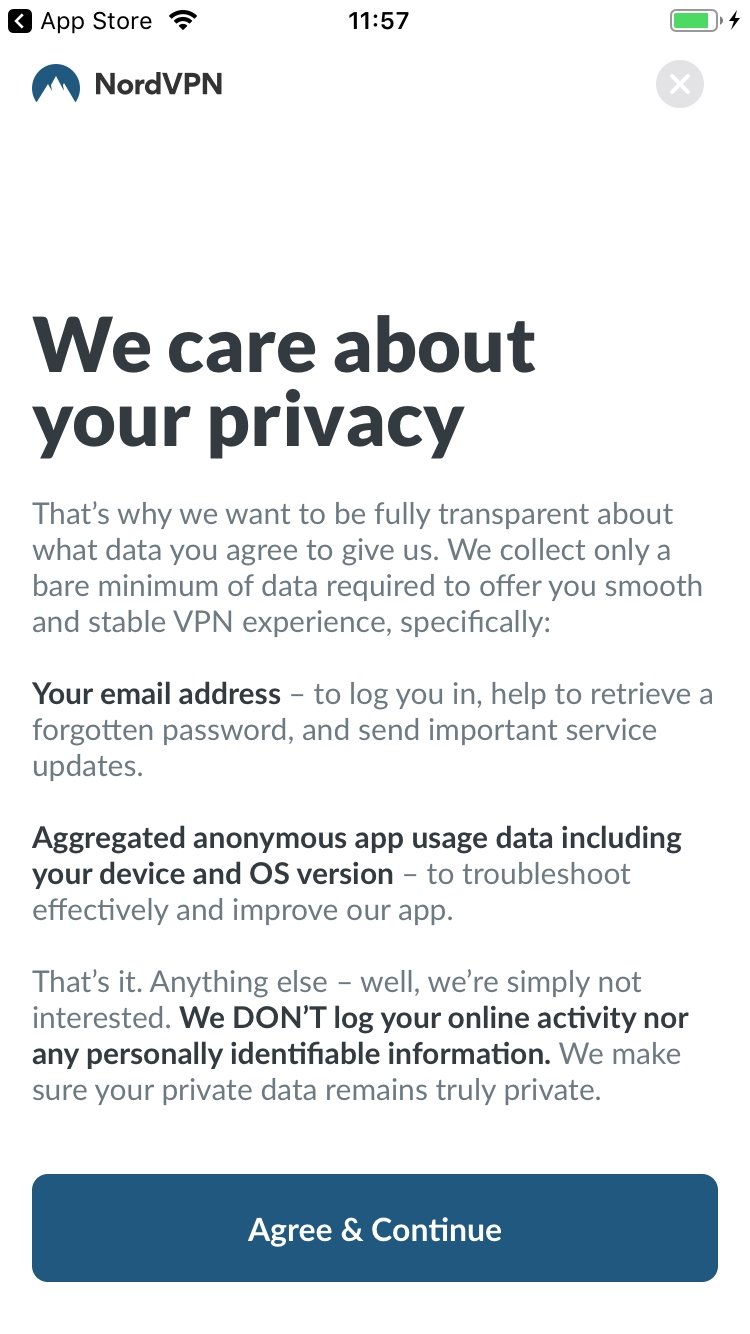The image shows the privacy notice for the NordVPN app, as viewed during its download from the App Store. At the top of the screen, it displays the App Store interface along with the current Wi-Fi connection status, the time (11:57), and a nearly fully charged battery that is connected to a charger.

Centered at the top of the notice, "NordVPN" is written in black letters alongside a graphic of a white mountain range set against a blue circle background. Below, bold black text states, "We care about your privacy." This is followed by a detailed explanation in smaller font, clarifying that NordVPN aims for full transparency regarding the data it collects.

The notice specifies that NordVPN collects only minimal necessary data: (1) your email address, used to log in, retrieve forgotten passwords, and send important service updates, and (2) aggregated anonymous app usage data, including device and OS version information, to troubleshoot and improve the app.

The policy emphatically states in bold letters, "We don’t log your online activity nor any personally identifiable information. We make sure your private data remains truly private."

At the bottom of the notice, there is a blue button with "Agree and Continue" written in white letters, inviting users to consent to the privacy terms.